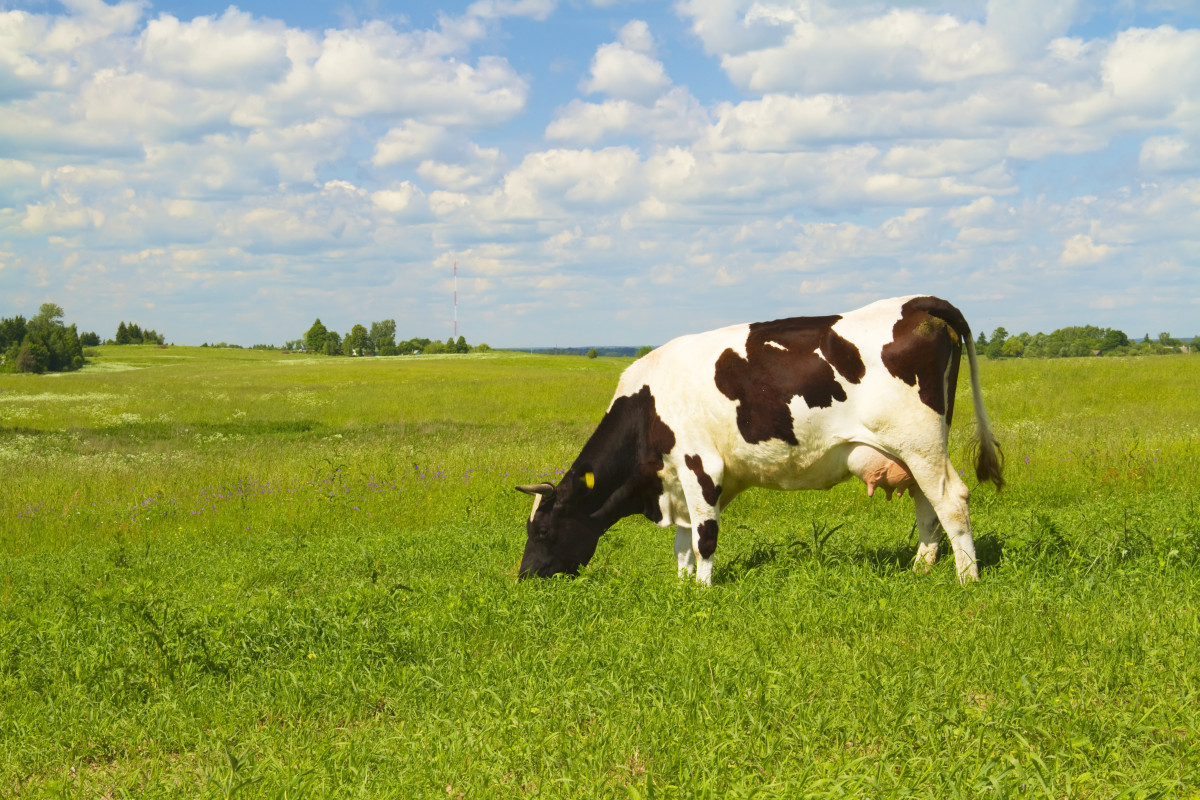This image captures a detailed scene of a lone cow grazing in a vast, grassy field during the daytime. The sky is a light blue adorned with large, pretty clouds, creating a serene backdrop that extends seemingly forever into the horizon. The field itself is expansive, filled with a mix of grass, weeds, and wildflowers that stretch back multiple acres. Distant clumps of trees and a few bushes dot the landscape. Far off on the horizon, an alternating orange and white cell phone tower can be seen.

The cow, a black and white milking cow with a stereotypical pattern, also features some light brown splotches on its front left leg and tail. It has short horns and is actively grazing, with its head buried in the grass. A yellow tag is visible on its left ear, likely for farmer identification. Seen from the left side, the cow's full udders indicate it is a milking cow, possibly having recently given birth. All four of its feet are firmly planted on the ground as it enjoys its meal in this idyllic, pastoral setting.